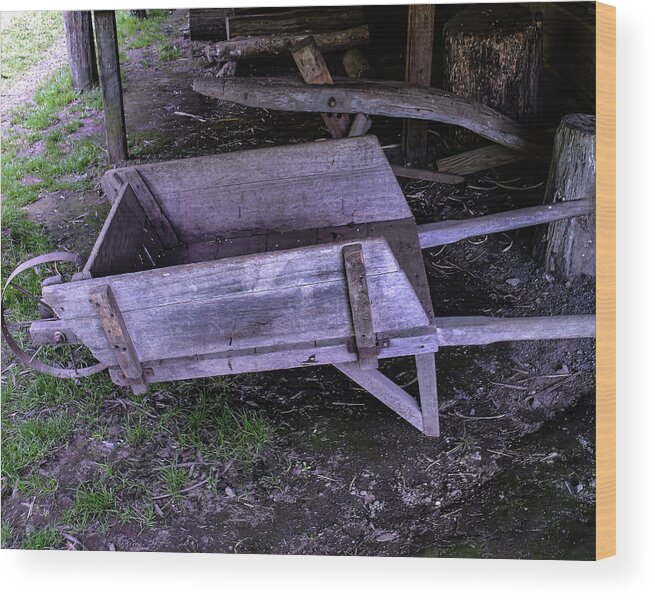The image depicts a highly detailed scene within a rustic, makeshift shed situated outdoors. The focal point is a weathered wooden wheelbarrow with a single metal wheel at the front, appearing old yet functional. The wheelbarrow's structure, including its base, handles, and support brackets, is entirely crafted from wood that looks dry and brittle. Surrounding the wheelbarrow, patches of green grass are sporadically scattered on the ground, which is predominantly dark dirt, appearing damp in some areas. The shed itself stands supported by aged, gray wooden posts, revealing a rugged and natural construction. In the background, piles of old, rotting wood contribute to the scene's rustic charm, alongside shorter logs and large wood stumps. The entire setting is characterized by a palette of grays, browns, blacks, and greens, emanating a sense of timeless utility and natural decay.